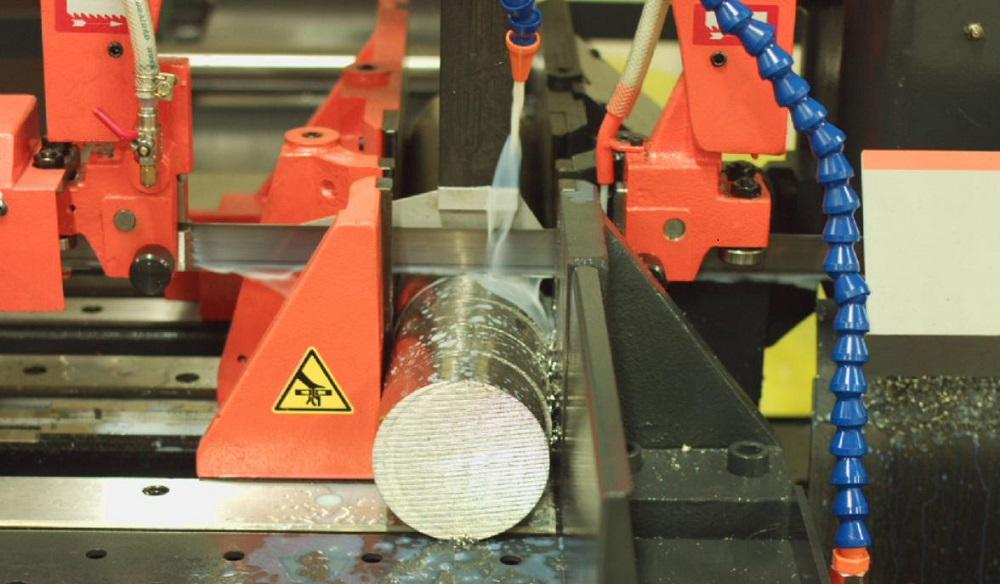The photograph captures a detailed view of industrial sawing equipment designed to cut cylindrical metal pieces. Prominent red clamps securely hold the cylindrical metal piece in place. Above this metal piece, a nozzle attached to a flexible blue tube dispenses a stream of white lubricant to keep the metal cool during the sawing process. Some of this lubricant has splattered onto the bottom center of the image and can be seen dripping from the metal piece. The machinery includes various metal and plastic components, as well as hoses that administer water to facilitate smooth cuts. A yellow triangular warning sticker on the equipment indicates the presence of a cutting blade, underscoring the equipment's purpose for making precise cuts in the metal.